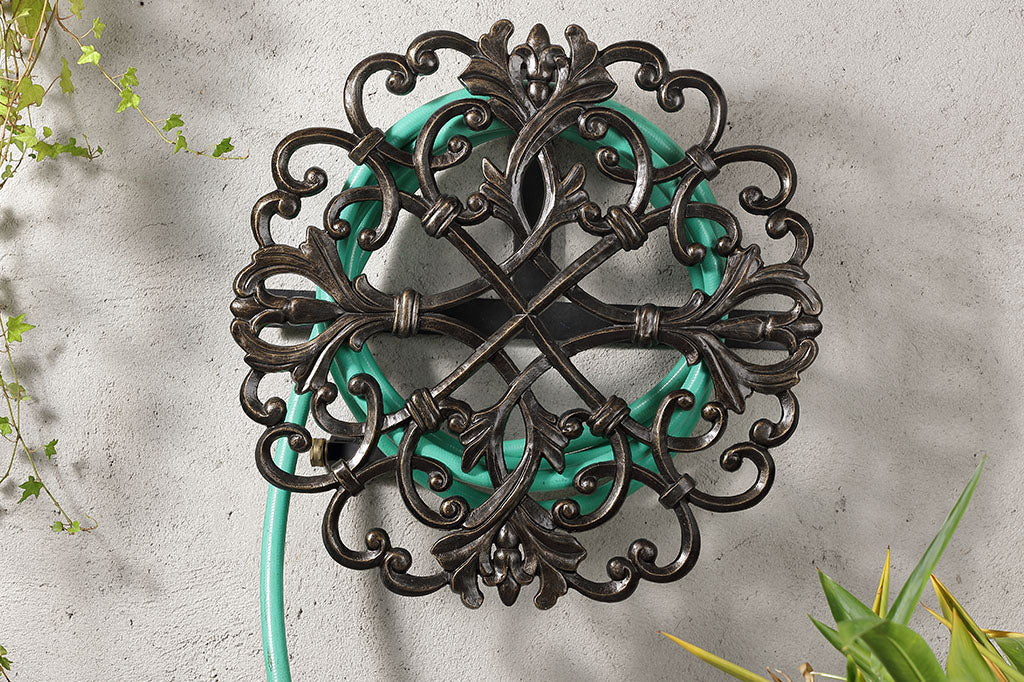This image features a beautifully ornate, vintage-inspired metal garden hose holder, crafted from black wrought iron. The intricate design showcases swirling, almost heart-like motifs encircling a central shape that resembles a four-leaf clover, lending an Irish-inspired touch. The hose holder is firmly affixed to a white concrete wall, and a vibrant teal green garden hose is neatly coiled around it, intertwining elegantly with the metal framework. To the left, a pothos plant climbs along the concrete wall, while a succulent or similar plant peeks out from the bottom right corner of the image. The composition, evocative of a stylish ad or a feature in a home and garden magazine or blog, underscores the functional yet decorative appeal of the hose holder in an outdoor setting.